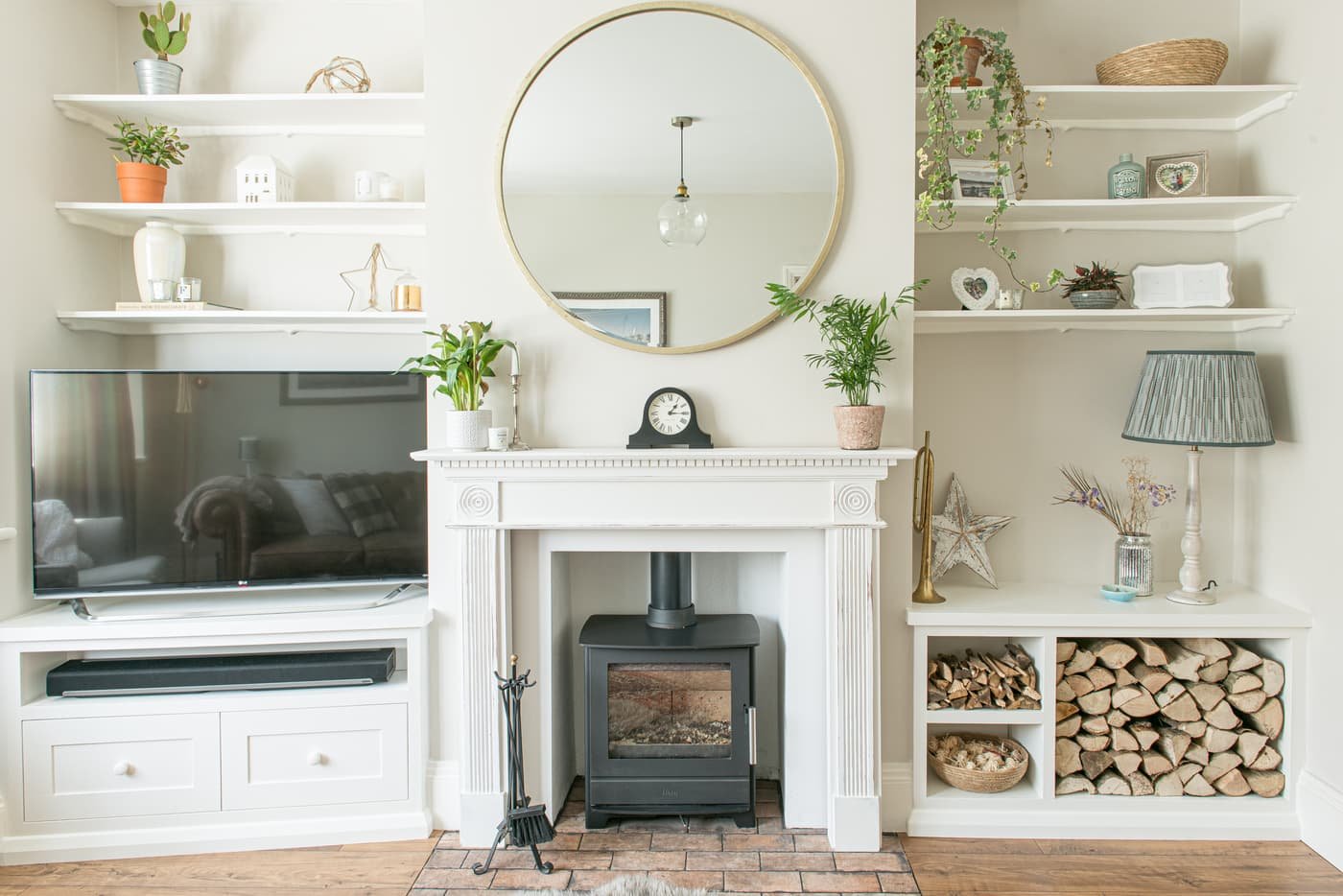This photograph captures a detailed and cozy living room wall, painted in light beige. Central to the composition is a white fireplace with a wood-burning stove inside, featuring a black metal stove and a pipe running up the chimney. The fireplace has a white mantle, adorned with a clock and two plants. Above the mantle, a large brass-framed mirror hangs, reflecting elements of the room including a chandelier and a picture frame.

To the right of the fireplace, there is a quaint nook with three white shelves at the top, each shelf adorned with decorative items. The top shelf displays a hanging plant with cascading leaves and a light-colored woven basket. The middle shelf holds a framed photograph, a heart-shaped frame with a picture, and a small blue bottle. On the bottom shelf, you'll find a white heart frame, a cat figurine, a potted plant in a gray pot, and a book sculpture. Below these shelves is an open cabinet filled with wood, topped with a white lamp with a green lampshade and a small silver vase containing flowers. Leaning against the wall next to this nook are an antique-looking star and a brass bugle.

On the left side of the fireplace is another similar nook with three white shelves at the top, each decorated with a plant. The middle shelf also holds a miniature house sculpture. Beneath these shelves is another white cabinet, housing a TV and a DVD player, along with two drawers at the bottom. The floor in front of the fireplace is made of brick, adding a rustic charm to the scene. Additionally, fireplace tools, including pokers and a brush, are placed next to the hearth, completing this inviting and well-organized living room setup.